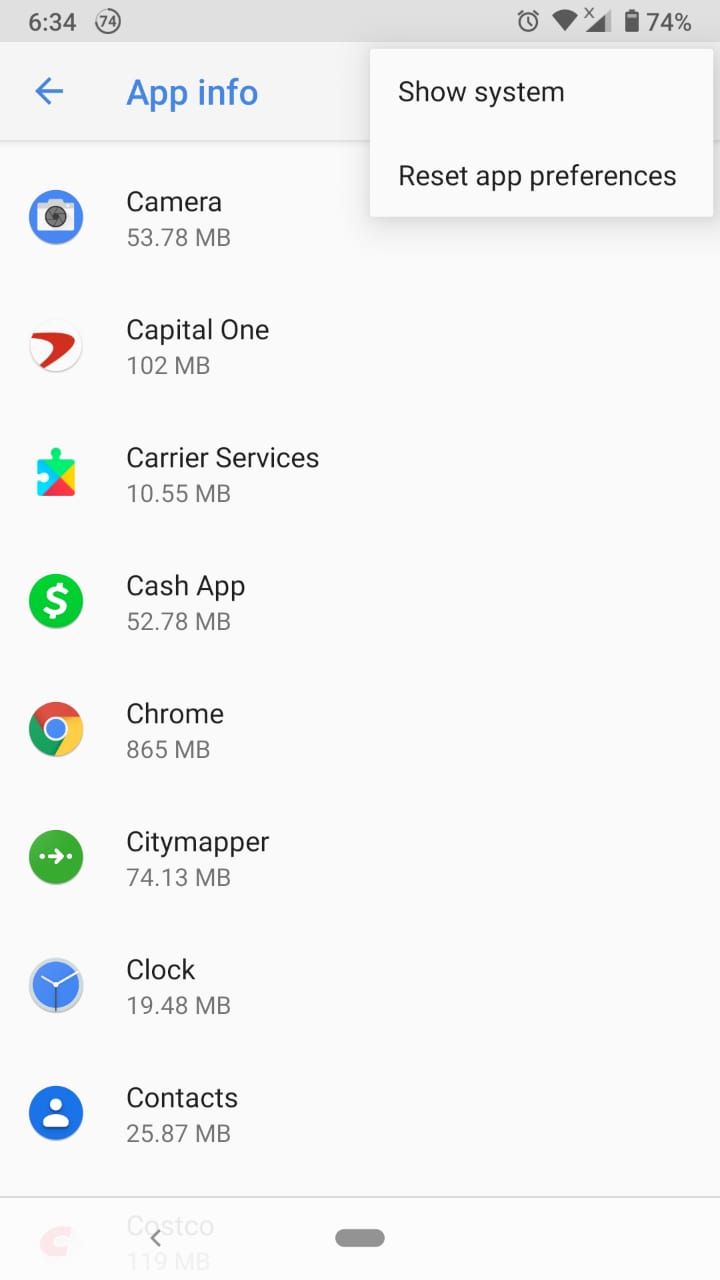A screenshot from a smartphone displays various app information. The time is shown at the top of the screen as 6:34 with the battery at 74%. Below the time, a gray area labeled "App Info" with a left-pointing arrow is present. The list of apps includes:

- **Camera** with an icon depicting a camera, using 53.78 MB.
- **Capital One** using 102 MB.
- **Carrier Services** using 10.55 MB.
- **Cash App**, indicated by a green circle with a dollar sign, using 52.78 MB.
- **Google Chrome**, noted with the Google icon, occupying 865 MB.
- **City Mapper**, marked by a green circle, using 74.13 MB.
- **Clock**, represented by a blue circle with clock hands, using 19.48 MB.
- **Contacts**, shown with a blue circle and a generic person icon, using 25.87 MB.

A small gray line runs underneath this list, likely indicating the end of the visible section.